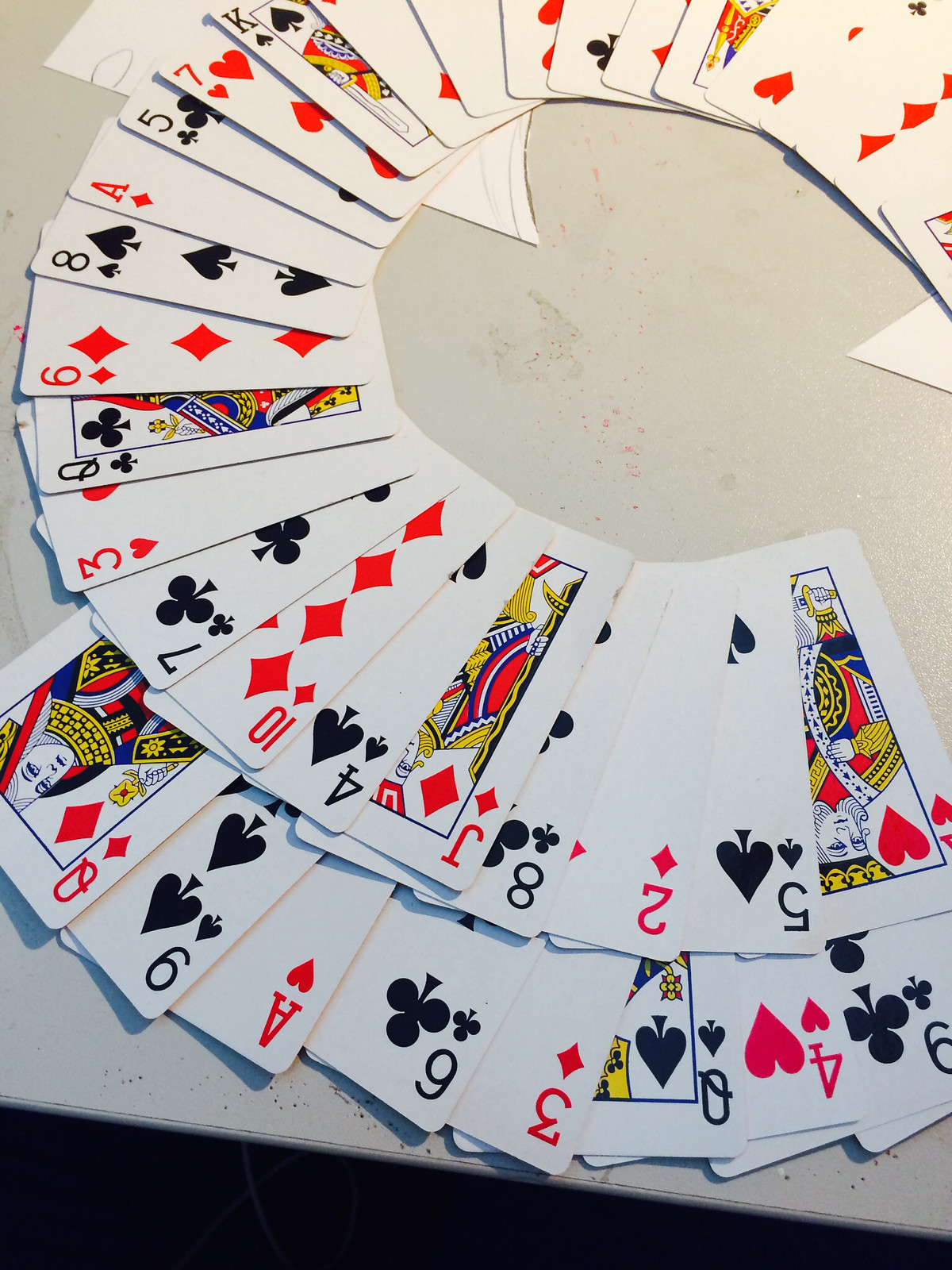The image depicts a complete deck of standard playing cards arranged in a circular pattern atop a gray surface. The circle, slightly incomplete with an eighth of its circumference open on the right side, is visually engaging and intricately detailed. The playing cards feature traditional suits—hearts, spades, diamonds, and clubs—rendered in classic black, white, red, and yellow hues. Among the cards are various numbered cards as well as face cards like kings, queens, and jacks, each designed with the iconic imagery associated with the suits. The cards start from the right side of the picture, spiraling outward, continuing around the top, and back to the right, creating a dynamic and artistic visual display.